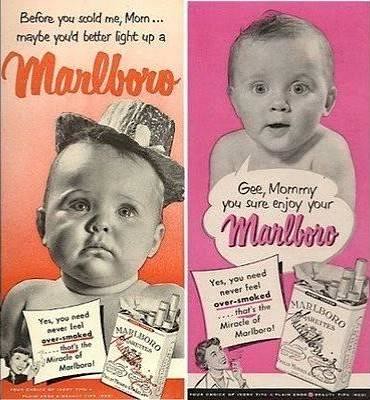This image is a peculiar, politically incorrect advertisement for Marlboro cigarettes from a bygone era. The ad is divided into two sections, each featuring a baby and a similar message extolling the virtues of Marlboro cigarettes. 

On the left side, set against a gradient background that transitions from orange at the top to red at the bottom, a black-and-white image of a baby wearing a hat and looking very sad is accompanied by the text: "Before you scold me, mom, maybe you better light up a Marlboro." Below, a drawing of a woman, presumably the mother, appears saying, "Yes, you need never feel over-smoked. That's the miracle of Marlboro," next to an illustration of the iconic cigarette pack with several cigarettes poking out.

The right side features a similar layout, but with a pink background. Here, a different baby, looking surprised and sad, has a speech bubble saying, "Gee, mommy, you sure enjoy your Marlboro." Again, a drawing of the mother, smiling while seemingly smoking a cigarette, says, "Yes, you need never feel over-smoked. That's the miracle of Marlboro," accompanied by another illustration of the cigarette pack.

The ad evokes a "very old-time" feel and starkly contrasts with today's advertising standards, highlighting its controversial nature due to the use of babies in promoting cigarettes.